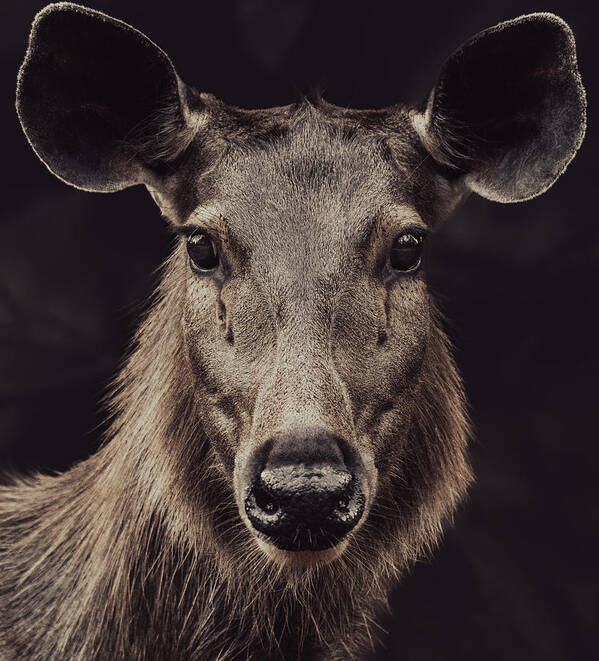This image is a detailed headshot of an animal resembling a deer, specifically a caribou or something similar, likely from a cold region. The animal is facing the camera directly with large, rounded black eyes that give an impression of a piercing stare. Tear lines are visible on its face, adding to its expressive look. It has a notably elongated muzzle and a solid black nose. The ears, which are perked up and somewhat oval-shaped, are lined in white, indicating adaptation to a chilly environment.

The fur on this animal is strikingly detailed, with a mix of brown, gray, black, and white shades giving it a textured and variegated appearance. The neck, in particular, is abundantly furry with long, somewhat straw-like hairs, contributing to its scruffy yet robust look. The coat transitions to slightly less dense fur toward its back. Notably, this animal lacks any antlers or horns, making the rounded ears more prominent in the composition.

Overall, the photograph captures the face and part of the neck of this intriguing creature, emphasizing its earthy color palette and the dense, varied fur texture that signifies its adaptation to colder climates.